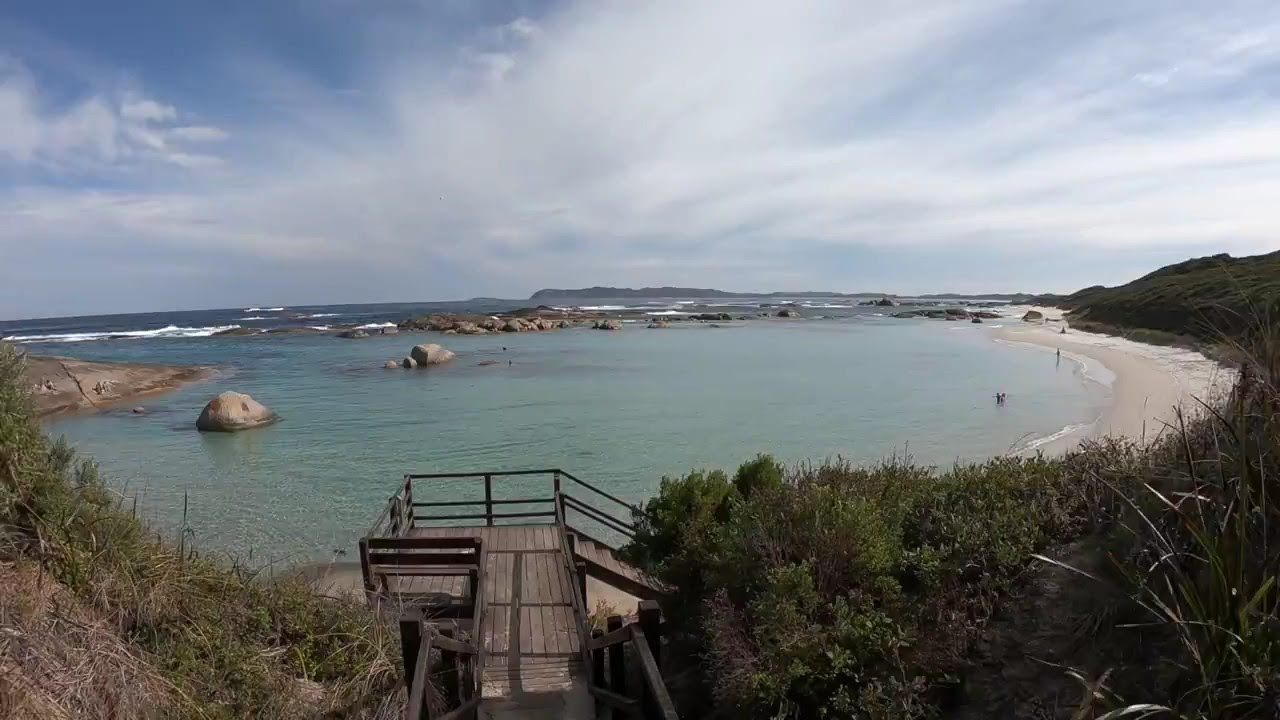The photograph captures a serene, slightly cloudy day at a public beach, viewed from an elevated vantage point. The scene showcases a circular-shaped bay enclosed by large rocky outcroppings to the left and verdant hilly terrain to the right. In the immediate foreground, a wooden walkway leads to a stairway that descends to the sandy shore, flanked by dry brush on both sides. On the beach itself, only a couple of people can be seen: one standing knee-deep in the water, and another with just a foot in. The vast, distant background reveals a large body of water, likely an ocean, bordered by green, grassy hills, and distant mountains. The entire coastline wraps around to the right, completing the tranquil setting.